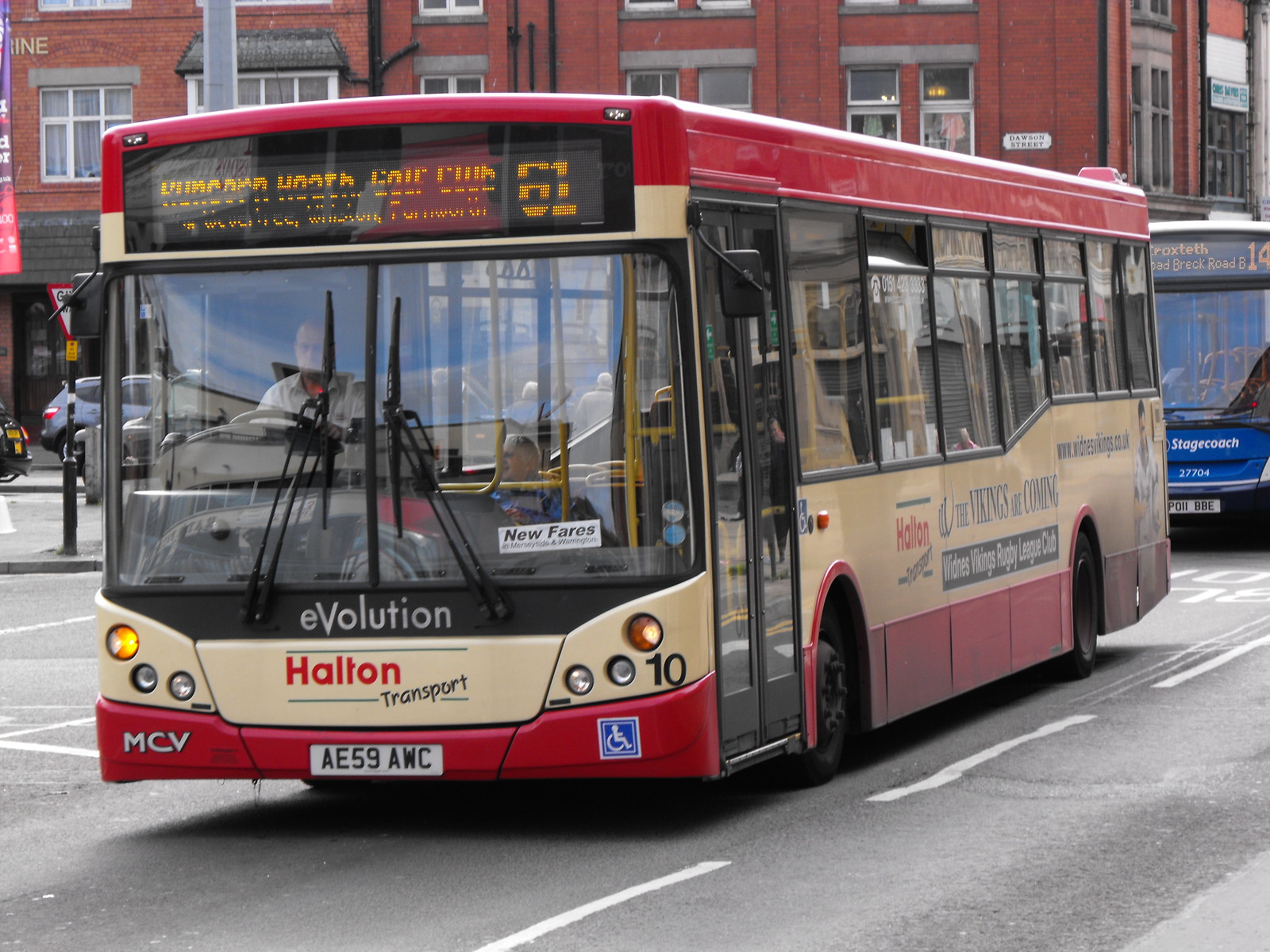The image captures a beige bus accented with a red top and bottom, traveling down a paved road marked by white dashed lines. The digital signboard at the front of the bus is broken and displays jumbled, incomplete letters, including the number "61." Below the windshield, the text "Evolution" is prominently displayed, followed by the company name "Helton Transport." The license plate reads AE-59AWC. MCV is marked on the lower left, and there is a handicap sticker as well with the number "10" above it. The bus features large side windows and a tall door, through which a faint image of the driver, dressed in a collared shirt, can be seen. Behind this bus, another bus, primarily blue, is visible. The backdrop includes a red brick building, adding to the urban setting of the scene.